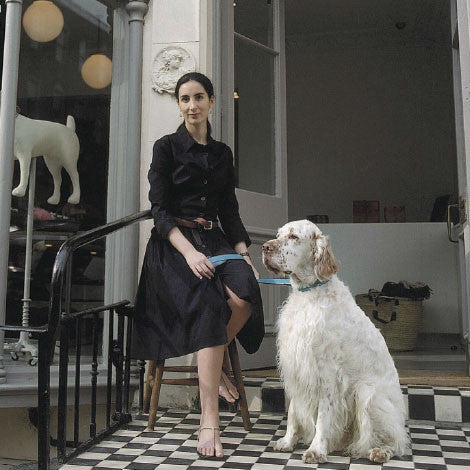In this colored photograph, a woman, seated outdoors on a stool, is positioned next to a black railing in front of a building with white, tall open doors. She wears a black dress cinched with a brown belt, and her feet are adorned with sandals. She holds a sky blue leash attached to a large, attentive white dog with brownish ears. The ground beneath them features a black and white checkerboard pattern. In the background, inside the open doors, there is a desk with a basket underneath, possibly containing clothes. Additionally, through a window on the left side of the building, part of a dog statue is visible.